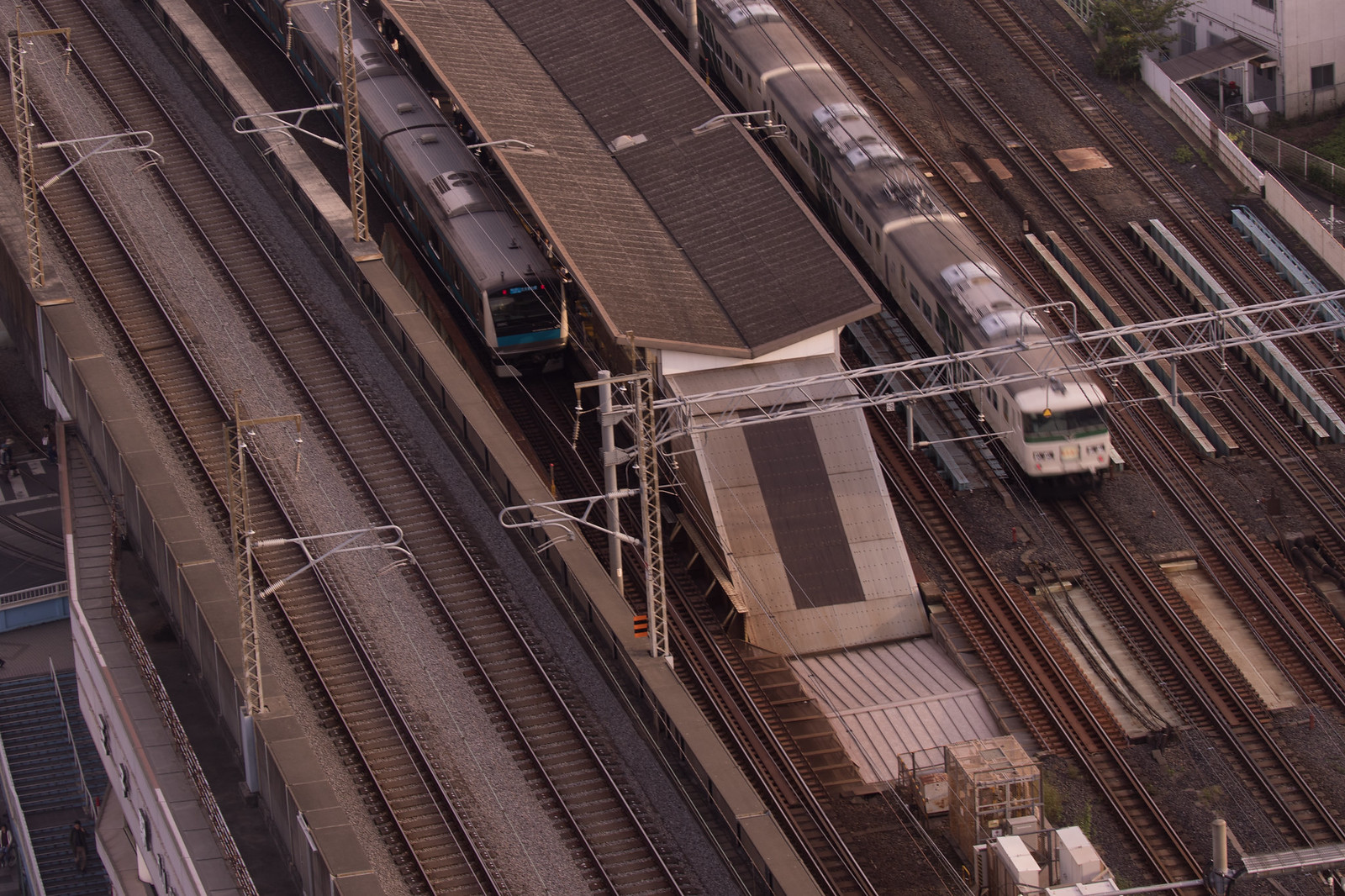This aerial image depicts a bustling train yard or elevated commuter railway station with numerous dark brown tracks, estimating at least eight or nine sets. At the heart of the scene is a main central platform, covered and raised, where passengers can board or disembark. Adjacent to this structure, there are two visible trains parked on either side. The left train features dark colors with hints of green, while the right one exhibits a white exterior with a gray top. To the right of the platform, a small building stands lower than the raised tracks. Steps on the far left descend from the elevated tracks, leading down to what appears to be a pedestrian access point. Overhead, sturdy posts and a structure reminiscent of monkey bars likely support electrical lines crucial for the trains' operation. The station is surrounded by additional empty tracks, emphasizing the scale and functionality of this transport hub.